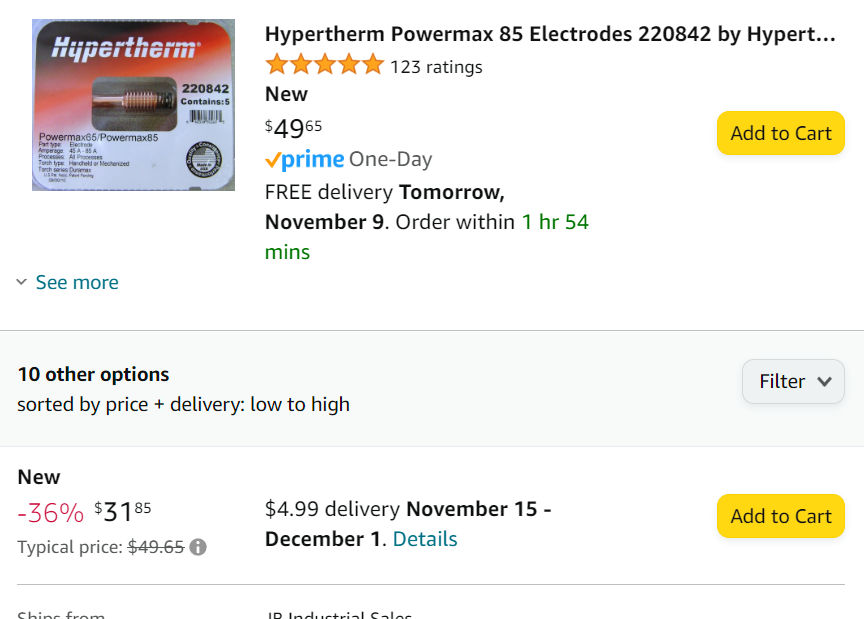This image appears to be a screenshot from Amazon, displaying a listing for Hypertherm Powermax 85 Electrodes (Model 220824). At the top left-hand side, there is a box featuring the Hypertherm logo on a white background, set against a red backdrop. Adjacent to this image, the product is listed as "Hypertherm Powermax 85 Electrodes 220824 by Hypertherm." The text trails off indicating it is truncated. The listing highlights a stellar five-star rating based on 123 reviews. 

The item is priced at $49.65 and is eligible for Prime One-Day delivery, offering free shipping with an estimated arrival of tomorrow, November 9. There is a prompt indicating customers should "Order within 1 hour 54 minutes" — this countdown is displayed in green text. A yellow "Add to Cart" button is prominently placed below this information, alongside a blue "See More" arrow on the left-hand side.

Just beneath this section, a light grey rectangle informs shoppers of additional purchasing options: "10 other options sorted by price plus delivery low to high," accompanied by a filter button on the right.

The next listed option showcases a new price tag of $31.85, reflecting a discount of 36%, down from the typical price of $43.65. It mentions a delivery fee of $4.99 with an estimated delivery window from November 15 to December 1. This option also has an "Add to Cart" button directly beneath it. There is a horizontal line under this button, partially obstructing the next segment of text, making it illegible.

Below this, there is an additional horizontal line separating further information that is cut off from the visible part of the screenshot.